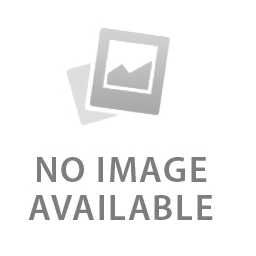The image features a packaged fridge magnet, prominently displayed in the center. The magnet, sealed in a clear cellophane bag, depicts a blue tuk-tuk taxi with a black roof, blue and pink striped seats with yellow trim, and a red, white, and blue striped flag on top. The taxi has "Taxi" written on it, and underneath the vehicle, it reads "I ♥ Bangkok" in black, with the heart in red. Behind the magnet within the packaging, a red background insert with a lighter pink flower is visible, and text in yellow reads "Magnet product of Thailand". The brand "Fridge M°" is also indicated. The packaged magnet, which has not yet been purchased, stands upright against a gray background.